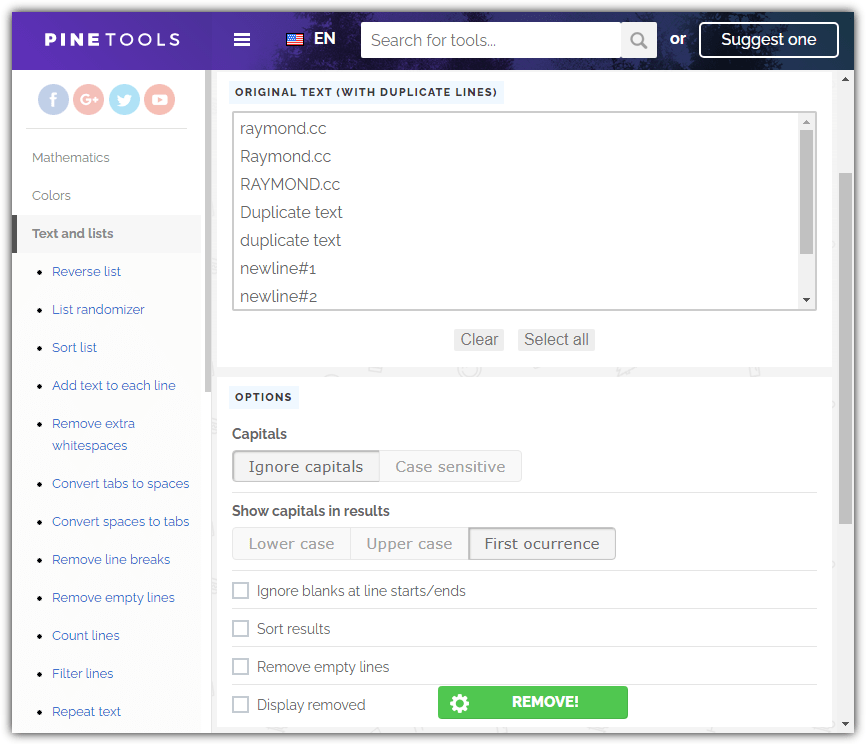This vertical image, which can be viewed on a computer, showcases the interface of a tool website. At the top, there is a purple-hued sky background with the website’s title "Pine Tools" in white. Adjacent to the title are three horizontal lines, denoting the menu for more options. An American flag icon indicates the English language preference.

In the background, the very tops of some trees are visible with their leaves creating a subtle backdrop. Below the header, there is a search box accompanied by a magnifying glass icon and a text instruction to "search for tools" or suggest one.

On the left-hand side, the interface features a white background with various social media icons for Facebook, Google+, Twitter, and Instagram. Underneath these icons, there are categories listed vertically in blue font with black bullet points, including "Mathematics," "Colors," "Text and Lists." Subcategories under "Text and Lists" follow, detailing various tools such as "Reverse Lists," "List Randomizer," "Sort Lists," "Add Text to Each Line," "Remove Extra White Spaces," "Convert Tabs to Spaces," "Convert Spaces to Tabs," "Remove Line Breaks," "Remove Empty Lines," "Count Lines," "Filter Lines," and "Repeat Text."

In the center, highlighted in light blue, the text "Original text with duplicate lines" is visible. Below this section, there is an area labeled "Raymond.cc" repeatedly with variations in capitalization (e.g., "Raymond.cc," "raymond.cc," "RAYMOND.CC"). Other options listed include "Duplicate text," "Duplicate test," and line numbers such as "New line number one" and "New line number two." 

There are buttons available for "Clear" and "Select All," separated by a grey line. A scroll bar is also present on the right-hand side for navigating. More sorting options are highlighted in light blue with uppercase text, including "Ignore Capitals or Case Sensitive," "Show Capitals in Result," and "First Occurrence" (currently highlighted).

Additional check options such as "Ignore Blanks," "That Line Starts/Ends," "Sort Results," and "Remove Empty Lines," remain unchecked. At the bottom right is a green "Remove" button, indicating an option to clear selected text or duplicates.